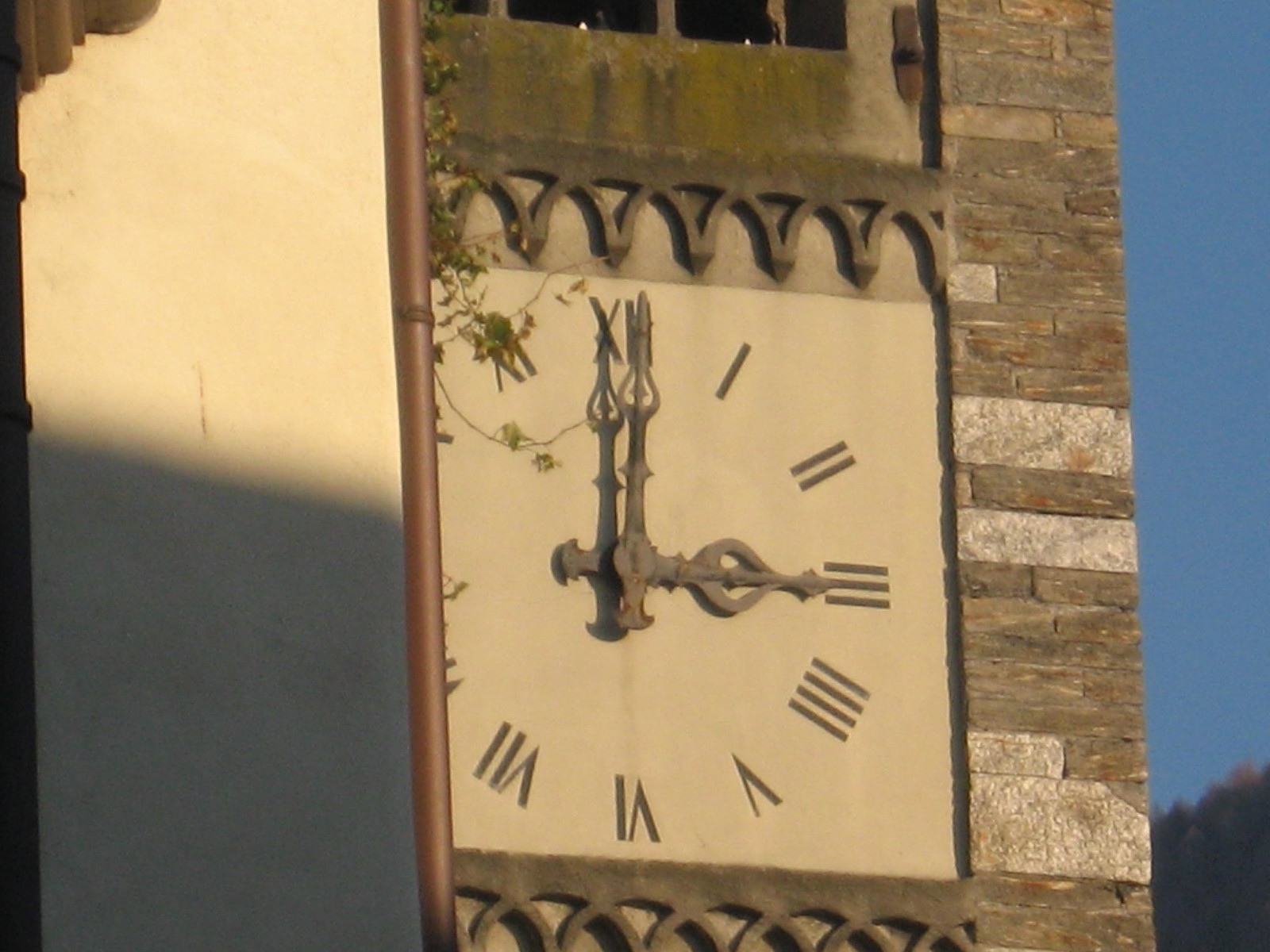A high-quality daytime photograph reveals a striking building facade adorned in shades of gray, brown, and tan stone. The sunlight reflects off the gray stone surface of the building, adding a subtle glow. To the left, a prominent terracotta-colored metal pipe contrasts against the stone. Dominating the right side of the image, an intricately etched stone clock with Roman numerals and grayish clock hands captures attention. Green leaves partially obscure the clock face, adding a touch of nature to the architectural scene. Below and above the clock face, darker gray stone carvings provide additional texture and detail. The building showcases a harmonious blend of various colored stones—brown, gray, and tan—creating an aesthetically pleasing and richly detailed composition.